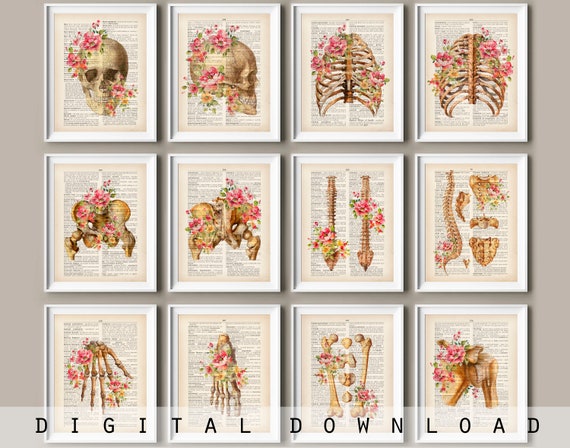This product image is a detailed digital download featuring a collection of 12 framed illustrations of various skeletal parts adorned with vibrant pink flowers and green foliage. The frames are arranged in a 4x3 grid against an off-white background resembling the pages of an old book with black text. Each skeletal component is intricately detailed:

1. The first row includes a front-facing skull with flowers blossoming from the eye sockets and a side-view skull similarly adorned with floral decorations.
2. The second row showcases the ribcage and its backside, followed by views of the pelvic bone from different angles.
3. The third row depicts the spine from both front and side perspectives, hand bones with floral accents, and foot bones similarly embellished.
4. The fourth and final row offers a detailed look at individual bones, including smaller bones and shoulder joints, also decorated with flowers.

At the bottom of the image, an opaque white banner features the text "digital download" in spaced-out black letters, indicating that these highly detailed, artistic prints are available for purchase.